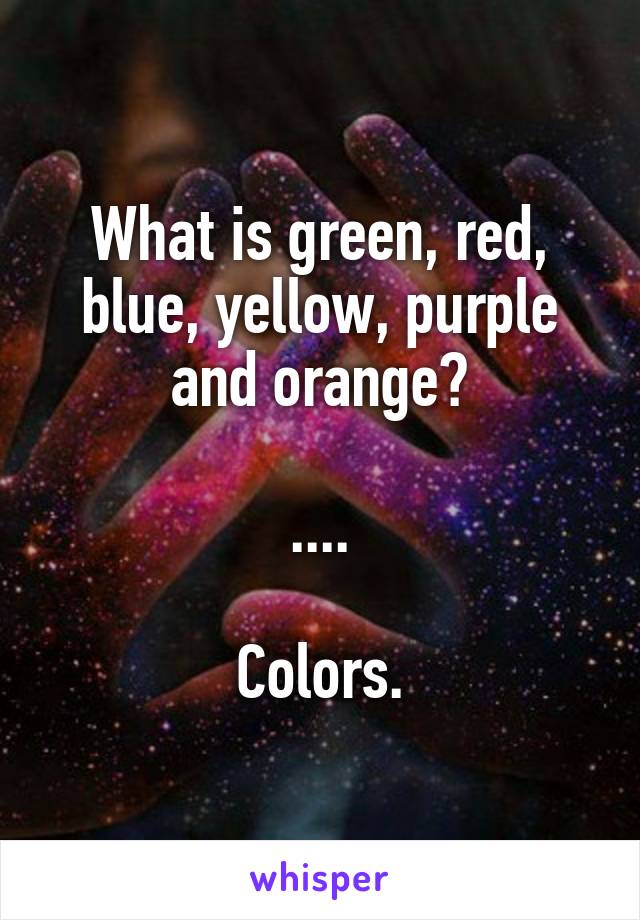The digital image showcases a surreal combination of text and cosmic elements. At the center, white text reads, "What is green, red, blue, yellow, purple, and orange?" Beneath this, a string of ellipses leads to the word "colors." In the background, a pair of hands stretch out, their fingers fanned and the palms darkened. These hands are adorned with galaxy-like imagery, rich in stars, with some stars glowing red and blue. The fingertips transition into more vibrant hues. A blurry visage, possibly a woman's face with brown hair partially covering it, can be seen faintly in the upper section. The overall scene is set against a dark backdrop, giving the composition a mysterious, cosmic feel. At the bottom, the word "whisper" appears in blue text on a small white rectangle, adding to the enigmatic tone of the image.